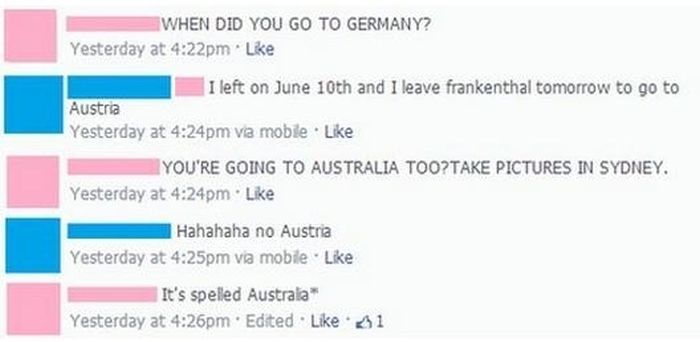Sure! Here's a cleaner and more detailed caption:

In this image, we observe a screenshot set against a white background. The screenshot features a pale lavender rectangle, containing a conversation. 

1. In the upper left corner, there's a pink square, followed by a bolded pink line of text that reads, "When did you go to Germany?" The timestamp for this question is "Yesterday at 4:22 PM." To the right of this, there's a word "like" written in a smaller font. 

2. Below, enclosed in a blue square, is the response: "I left on June 10th and I leave Frankenthal tomorrow to go to Austria." This response is in light lavender text and is timestamped "Yesterday at 4:24 PM via mobile."

3. Just below this, the pink square responds in capital letters: "YOU'RE GOING TO AUSTRALIA TOO? TAKE PICTURES IN SYDNEY." This light lavender text is timestamped "Yesterday at 4:25 PM via mobile."

4. Subsequently, the blue square replies, "Ha ha ha ha, no Austria," with the same light lavender timestamp design, "Yesterday at 4:25 PM via mobile."

5. Finally, the pink square makes a follow-up comment: "It's spelled Australia," posted at "Yesterday at 4:26 PM" and this comment has garnered one like.